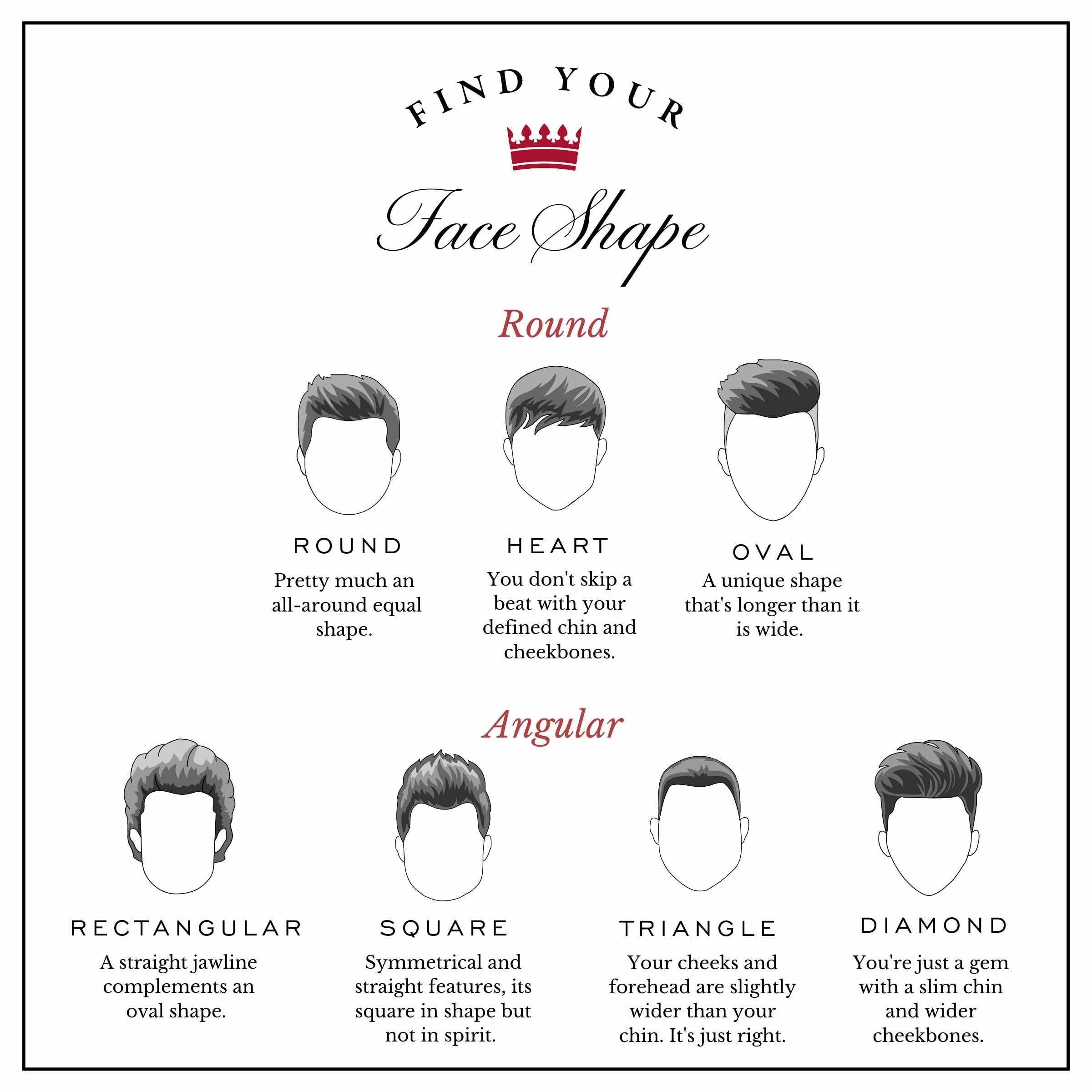This image features a detailed chart titled "Find Your Face Shape," which is presented in an italic font with the words "face shape" rendered in cursive. Between "find your" and "face shape," there's a small red crown logo. The chart categorizes different head shapes into two main sections: "Round" and "Angular."

In the "Round" section at the top, three different head shapes are listed: round, heart, and oval. Each head shape is just an outline without facial features, accompanied by a brief description underneath. For example, the round shape is described as "an all-around equal shape" and the heart shape is noted for a "defined chin and cheekbones."

The "Angular" section at the bottom includes four head shapes: rectangular, square, triangle, and diamond, each with its own description. Rectangular heads have a "straight jawline complements an oval shape," square heads are "symmetrical and straight features," triangle heads have "slightly wider cheeks and forehead than the chin," and diamond heads are "a gem with a slim chin and wider cheekbones."

All the head shapes are depicted with various black hairstyles, though the focus is on the head shapes rather than the hairstyles themselves. The overall coloring of the chart is white, allowing the black outlines and red crown logo to stand out prominently.